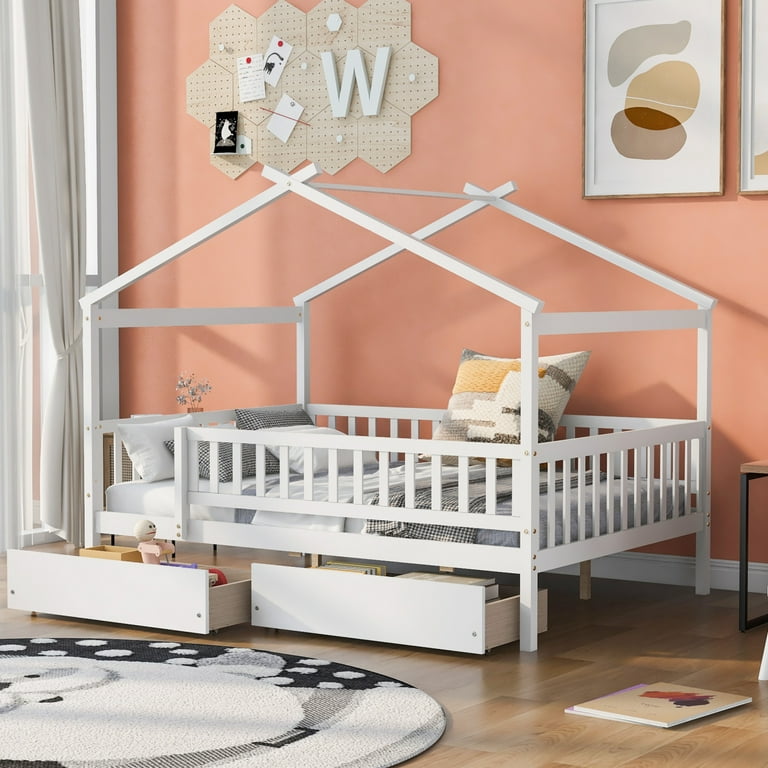The photograph captures a cozy and whimsically designed children's room. Central to the scene is a distinctive white wooden bed, equipped with a secure fence that wraps around it, leaving a small entry point for easy access. The bed is adorned with a white and black buffalo check bedspread and small pillows, lending a touch of classic charm. Beneath the bed, two drawers, partially pulled out, are brimming with books and toys. 

Adding to the bed's unique appeal is an unfinished peaked roof frame, hinting at a playful house-like canopy. The room's soft salmon or peach-colored walls create a warm background, contrasted by an array of artistic elements. To the upper right of the wall, framed artworks add a splash of creativity, while to the upper left, a hexagonal pegboard offers functional charm with its patchwork design and a prominent 'W'. 

In front of the bed, there's a black and white geometric rug featuring diverse patterns including circles and stripes, setting a striking visual base on the glossy laminate wood floor. The floor's edge is lined with crisp white baseboards, enhancing the room’s polished look. A large full-length window draped in white curtains on the left side fills the space with natural light, completing this inviting and thoughtfully decorated child's sanctuary.